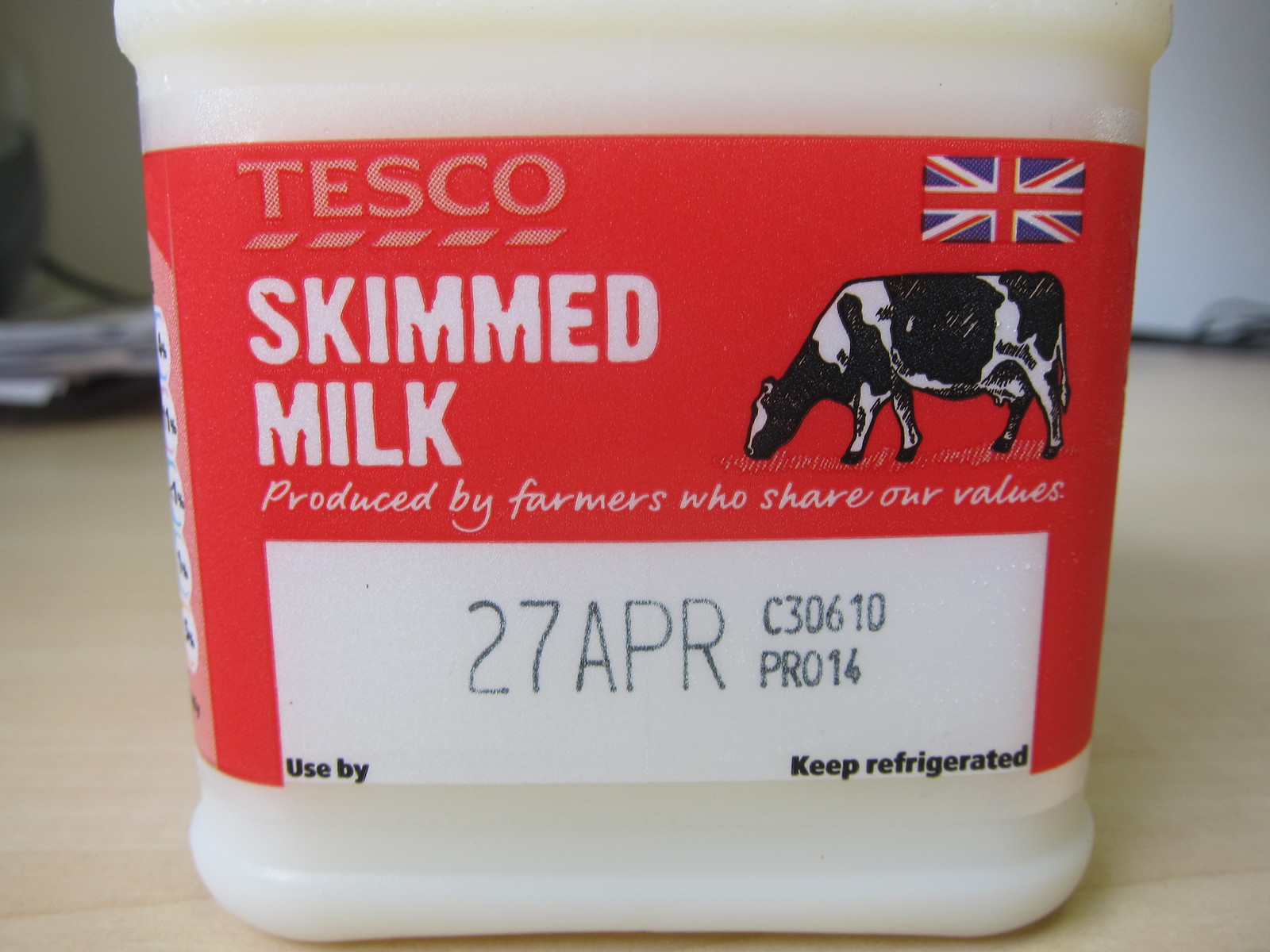This image features a short, squat plastic bottle of Tesco Skimmed Milk. The bottle, which has a somewhat cube-like shape, is only partially visible from the bottom to the label, with its clear plastic body showing the white milk inside. The label is predominantly red and white, wrapping around the circumference of the bottle. On the upper left of the label, it reads "Tesco Skimmed Milk," and on the upper right, there’s a British flag. Below the flag is an illustration of a black and white spotted cow grazing on grass. Beneath the cow, in white cursive text, it states "Produced by farmers who share our values." There’s also a large white rectangular box on the label containing the expiration date, "27 April," along with additional information and codes, "C30610" and "PRO14." The instructions "Use by 27 April" and "Keep refrigerated" are also clearly visible.